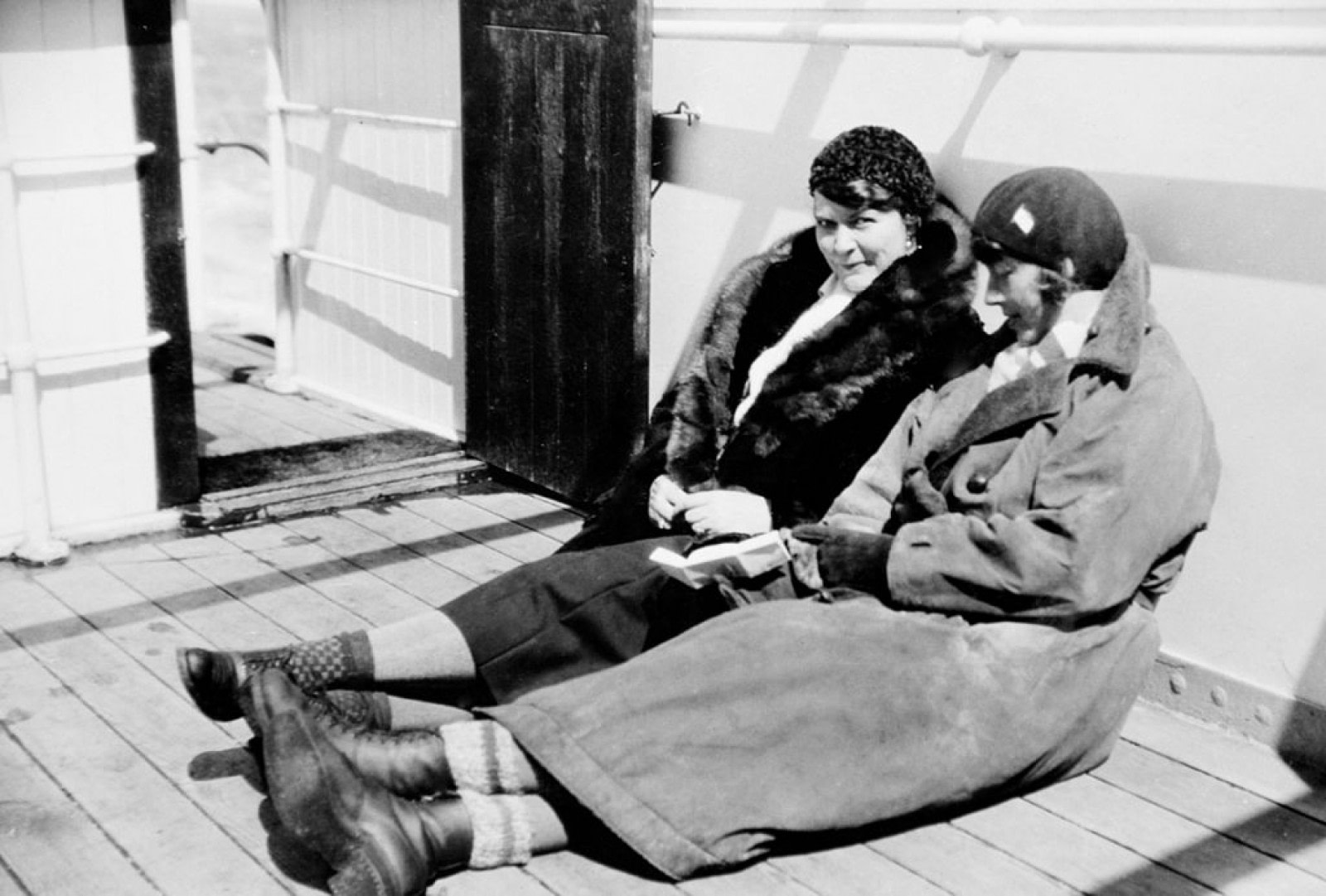This black and white photograph from the 1920s to 1940s captures two women sitting on a wooden deck outside, leaning against a white wall in the cold. Both are dressed for the weather in thick, dark-colored coats, winter hats, socks, and boots. The woman on the left, wearing a coat with fur edges, has a scarf and is looking directly at the camera, while the woman on the right, with gloves, looks down at her hands. Shadows suggest it's a sunny day. To their right, an open black door reveals a white interior wall. Above them, a white pipe-like structure is attached to the wall, adding to the aged ambiance of the scene.